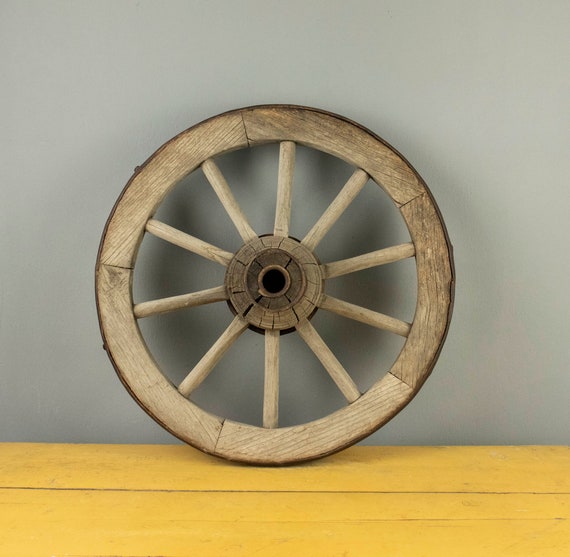The image depicts a vintage wooden wagon wheel leaning against a plain gray wall, casting a slight shadow. The wheel, made of pine wood and showing signs of age and mild weathering, consists of a circular outer rim reinforced with a metal band and a central hub with a small hole. Extending from the hub to the outer rim are ten round wooden spokes, arranged in a V pattern. The floor beneath the wheel is made of yellow pine wood planks, possibly painted, creating a striking contrast with the gray wall. The wheel is positioned upright on these planks, emphasizing its rustic charm and highlighting its detailed construction.